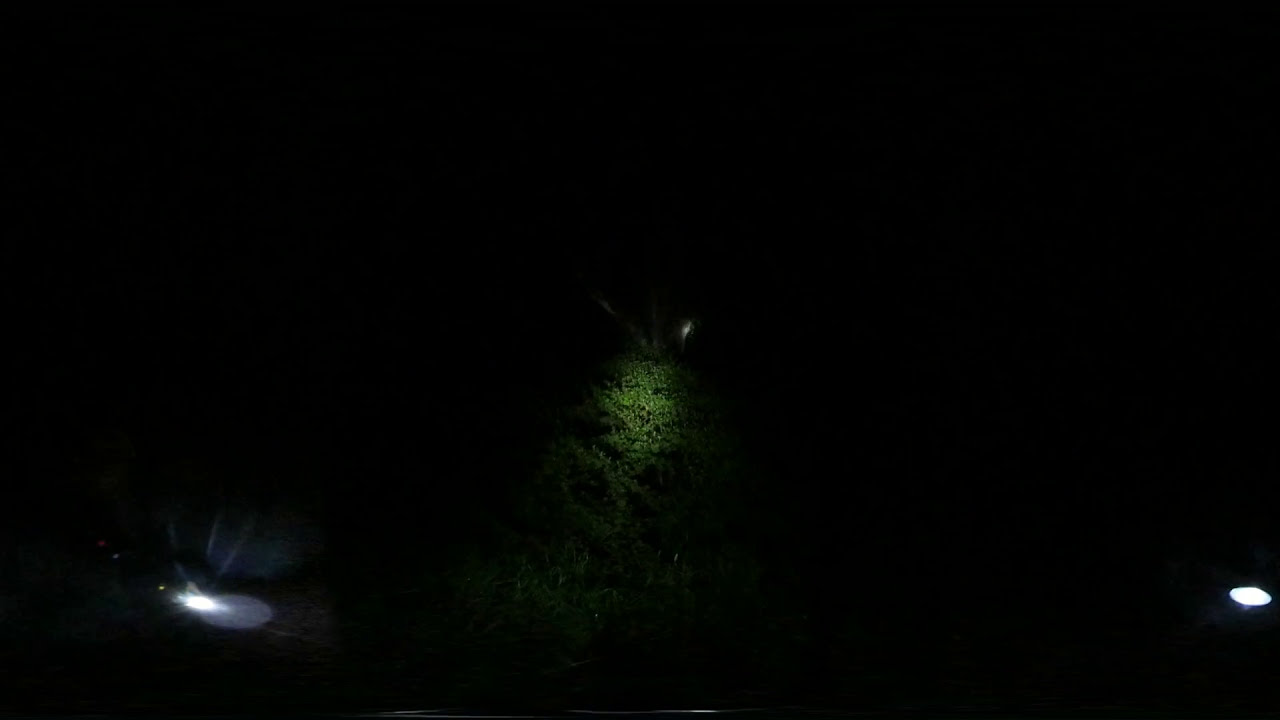This photograph is an overwhelmingly dark, nighttime outdoor scene, with 98% of the image in deep blackness. The sparse illumination in the image is noteworthy. In the bottom-left corner, there is an orb of light, possibly from a flashlight or lamppost. Similarly, another orb of light is present in the bottom-right corner. The central focus is a small but discernible green tree or tall bush, which appears almost to be glowing due to an artificial light source directly above it. The leaves and the faintly visible ground are gently bathed in this light, enhancing the tree's visibility against the dark backdrop. Additionally, there is another light positioned above and somewhat behind the tree, casting a soft illumination around it. The overall stillness of the scene hints at a peculiar, eerie atmosphere.